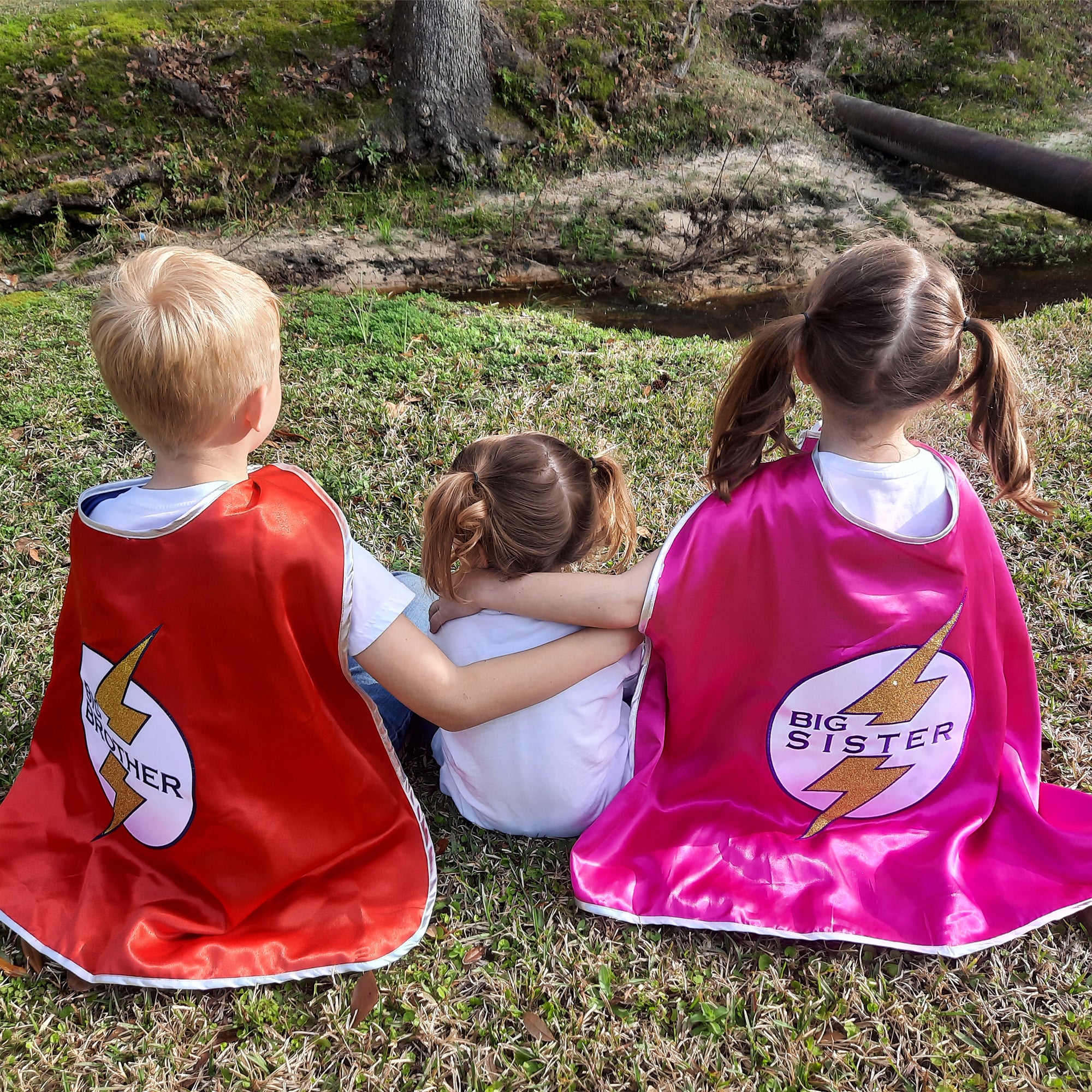The photograph captures a poignant moment of three children sitting together on the grass, facing away from the camera, with a small creek and a pipe visible in the background. The young boy on the left sports a red cape emblazoned with "Big Brother" and a lightning bolt, and he has blonde hair. The middle child, a younger girl with light brown hair in pigtails, wears a white t-shirt. To her right, an older girl also with light brown hair in pigtails wears a pink cape that says "Big Sister" with a lightning bolt. Both the older brother and sister are seen lovingly wrapping their arms around their younger sister, all dressed in white t-shirts, creating a heartwarming family scene highlighting their close bond.